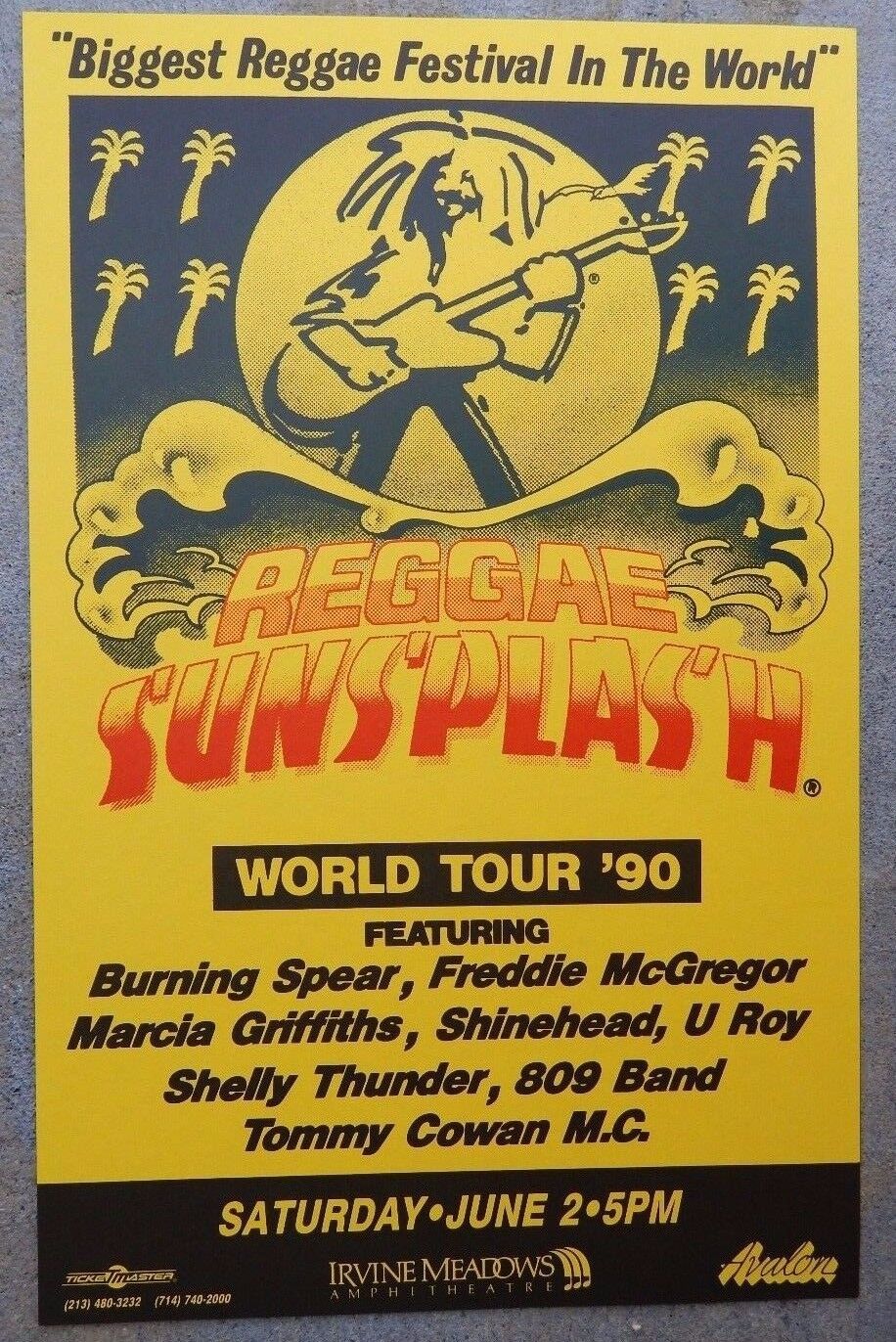This vintage Reggae Sunsplash poster from the 1990 World Tour is predominantly yellow with striking red and black text. Touted as the "Biggest Reggae Festival in the World," the poster features a prominent image of a dreadlocked guitarist playing energetically against a backdrop that includes palm trees and a wave crashing forward. The event is headlined by renowned artists including Burning Spear, Freddie McGregor, Marcia Griffiths, Shinehead, U-Roy, Shelly Thunder, 809 Band, and Tommy Cohen MC. Additional details include the date and venue: Saturday, June 2nd at 5 p.m. at the Irvine Meadows Amphitheater. Despite its simple, cartoon-like design, with a monochromatic palette aside from the vibrant text, the poster captures the essence and vibrancy of reggae culture from that era.